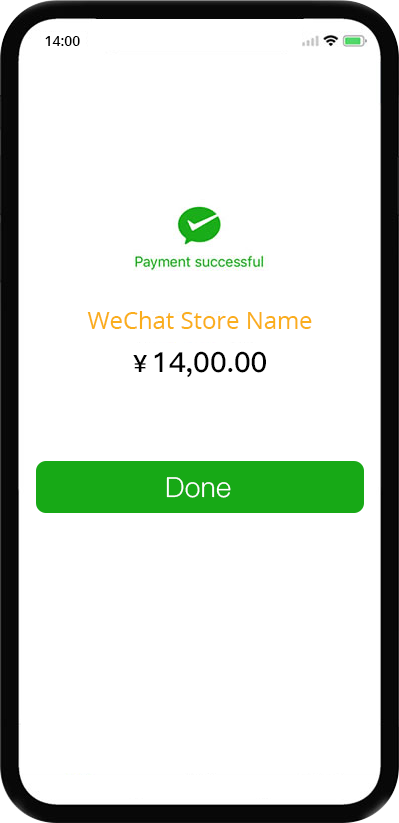The image depicts a phone screen with various interface elements. In the top left corner, the time is displayed as "14:00." On the top right, three icons are visible: a service bar indicator, a Wi-Fi symbol, and a battery percentage icon. 

The main section of the screen features a predominantly white background. At the top center, within a green thought bubble, there is a prominent checkmark accompanied by the text "Payment Successful." Below this, the name "WeChat Store Name" appears in orange. 

Still centered, the next line shows a currency symbol followed by the amount "14,000.00." Further down, within a green rectangular button, the word "Done" is displayed. The rest of the background remains completely white, drawing attention to the text and elements in the middle of the screen.